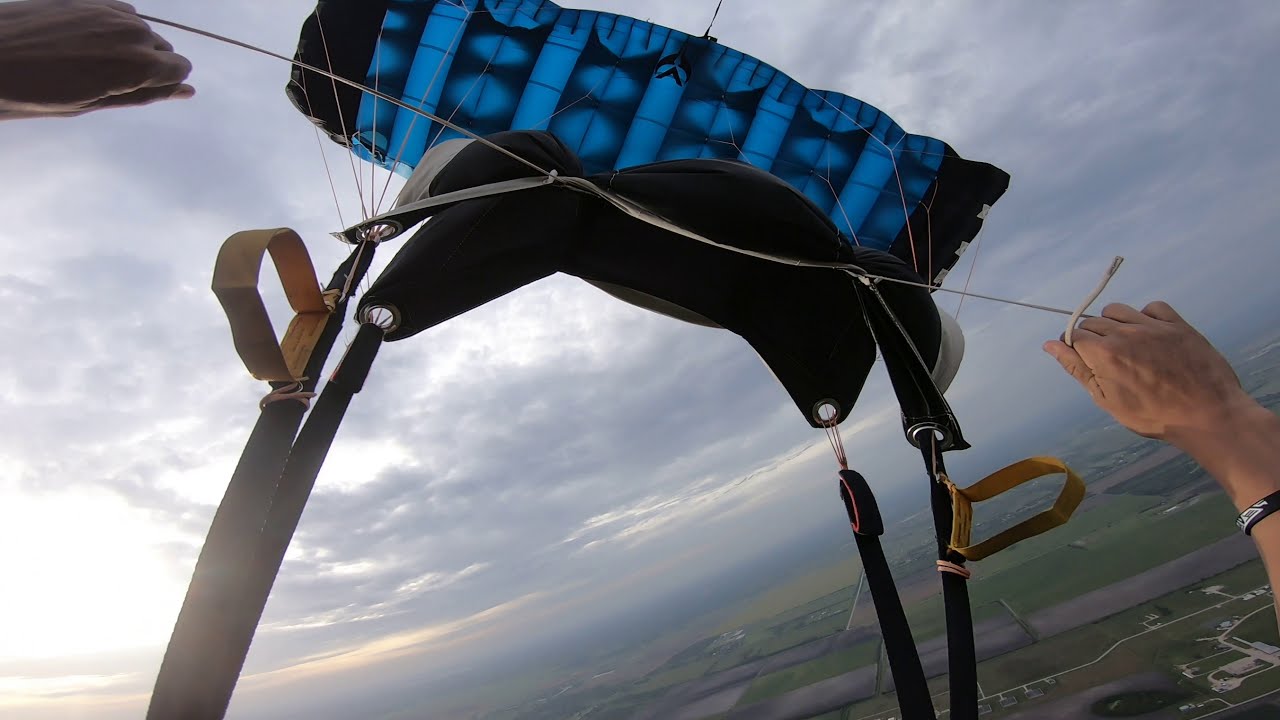The image captures a close-up of someone navigating a rectangular parachute, suspended high in the air. The parachute, which features a striking pattern of navy blue and sky blue stripes interspersed with diamond shapes, dominates the upper portion of the frame. Both hands of the parachutist are tightly gripping the control ropes: a brown hand hold on the left and another hold on the right. The ropes are connected to a harness made of dark material, with some straps appearing yellow and tough. The sky above is cloudy and predominantly gray, creating an overcast but daytime atmosphere. Below, the landscape features patches of greenery interspersed with farms, small houses, roads, and some distant structures, suggesting a rural setting.